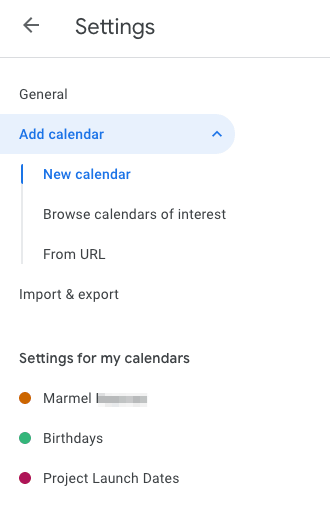The image displays the settings page of a calendar application. At the top of the page, the word "Settings" is prominently written in black on the menu bar. Below "Settings," the options "General," "Add Calendar," and "New Calendar" are listed, with "Add Calendar" and "New Calendar" highlighted in blue.

Underneath these options, a list of additional settings appears in black text: "Browse calendars of interest," "From URL," "Import," and "Export." Following these options, the section "Settings for my calendars" is displayed, featuring three specific calendars, each differentiated by a colored circle to the left of their respective names. The first calendar is named "Mamel," represented by an orange circle. The second calendar, "Birthdays," is marked with a green circle. The third calendar is "Project launch date," denoted by a maroon circle.

The entire background of the image is white, providing a clear contrast to the black text and colored elements. The layout emphasizes the functional organization of the settings page, ensuring that all text and icons are easily readable.